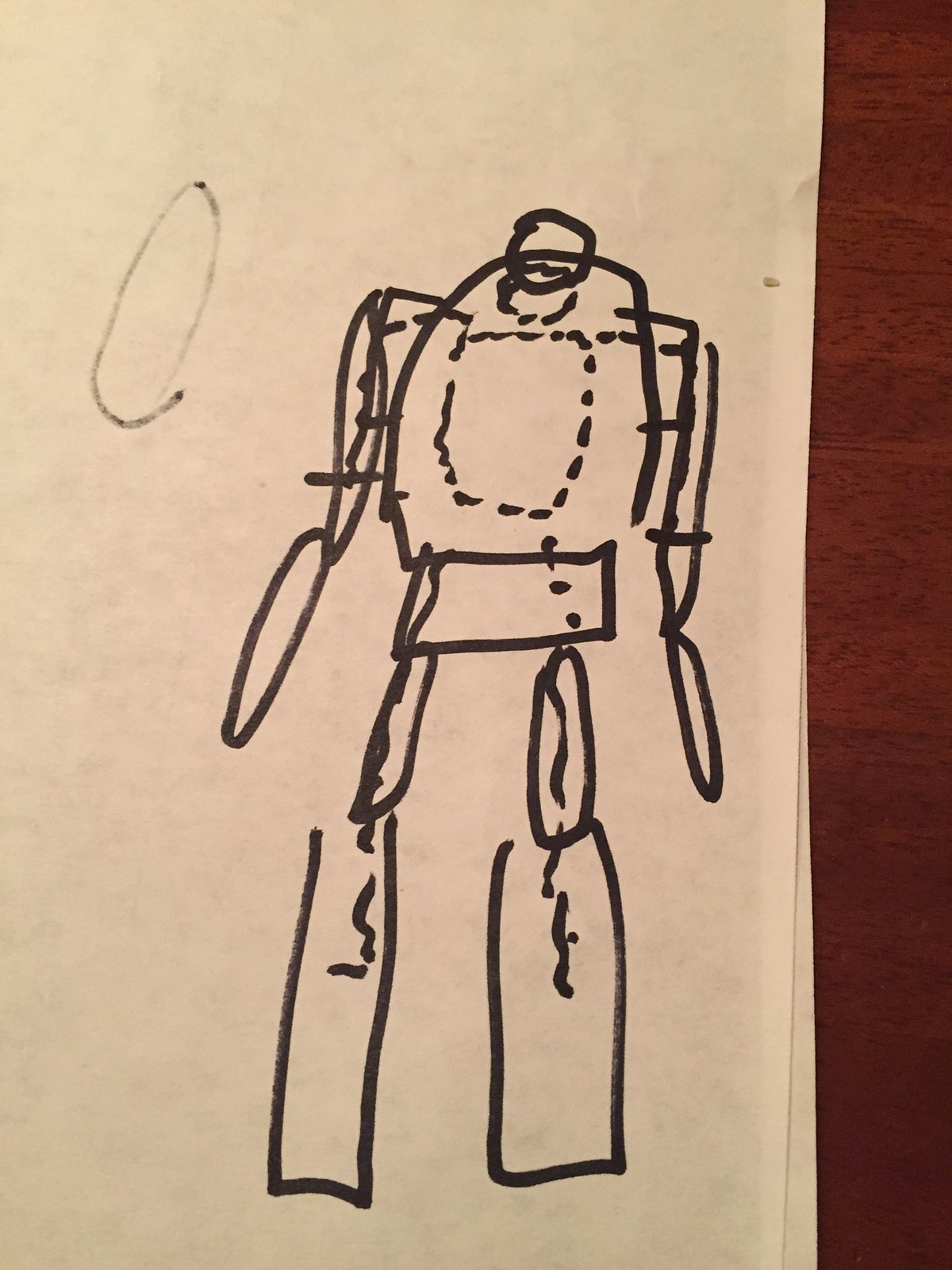This is a detailed marker drawing of a robot on a slightly faded yellow piece of paper, which lies on a reddish-brown wooden table. The robot has a small round head and a semi-round body. Its arms are thin lines ending in elongated circles. The robot's pelvis is rectangular, leading to thick, oblong upper legs and long, rectangular lower legs, both featuring black lines down the center. The robot's dotted square chest and neck, as well as the dots running down the right side of its pelvis, emphasize its mechanical nature. To the far left of the image, there is an additional black marker circle, with parts of the diagram appearing faintly as if they are bleeding through from the other side of the paper.